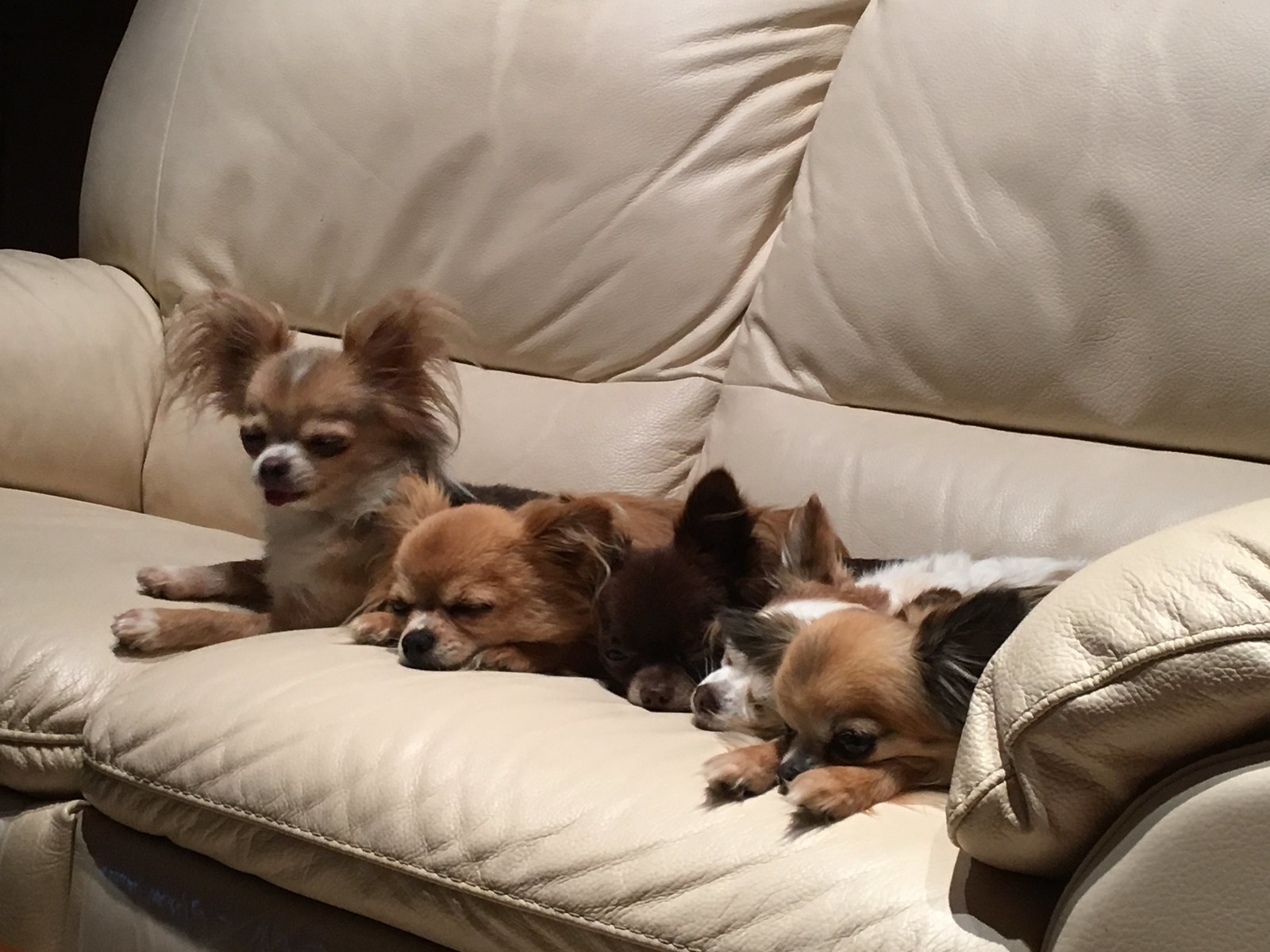This enchanting photo captures a snug gathering of six tiny chihuahua mix puppies, dozing on a plush white leather love seat. The love seat stretches from right to left, with the backrest gently inclining upward. The puppies, each weighing around five pounds, display a spectrum of colors: several are shades of brown with variations from light sable to deep chocolate, a couple feature white fur, and one is distinctly black with white markings.

Five of the puppies appear deeply sleepy, their eyes closed or partially shut, while one on the far left sits alert, its fluffy, ear-fanned head raised. This attentive puppy is a light brown with long, curly fur. Beside it are more brown-colored siblings, each nestled close together. Notably, there's also a nearly all-brown puppy, a predominantly white one with dark accents around its face and ears, and the unique black puppy, whose little face and ears peek out from the cozy pile. Each pup looks irresistibly cute, with characteristic traits of long-haired chihuahuas such as soft, wispy ears and striking black eyes, creating an adorable and heartwarming scene.